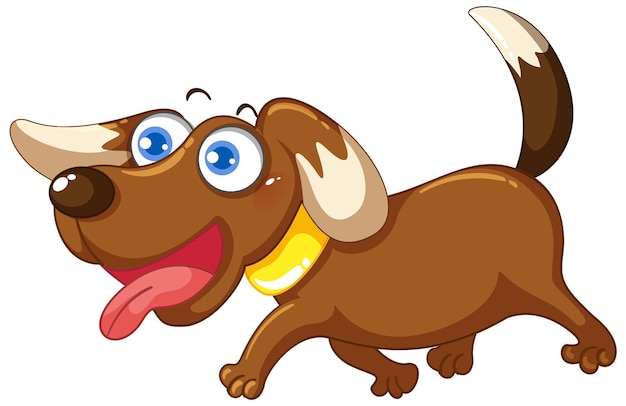The image is a detailed, cartoon-style illustration of a brown dog that resembles a Dachshund. The dog is depicted in a simple line drawing style with block coloring. It is primarily a deep rusty brown with a slightly darker brown tail that features white highlights on its tip and ears. The dog is centered in the image, looking to the left with its mouth wide open, revealing a dark pink interior and a light pink tongue with highlights. The dog's nose is a circular, dark brown with some black shading. Above its intense, large blue eyes are small, crescent-shaped eyebrows. The dog wears a golden collar with distinct colored highlights. While appearing to pant and walk, the dog’s long ears hang down on each side, further adding to its expressive and playful demeanor.